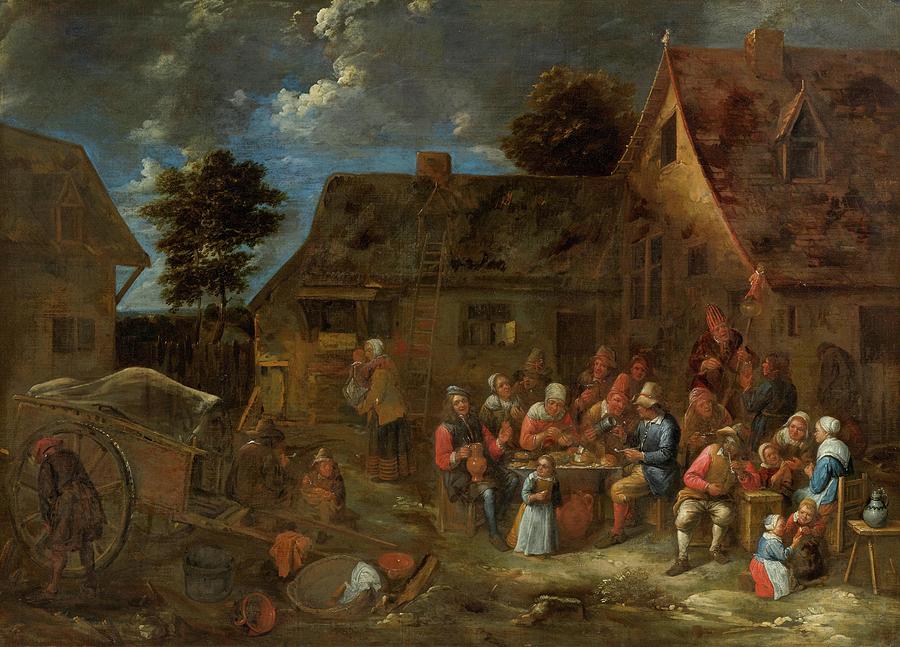This rectangular painting, measuring roughly six inches wide by four inches high, is an old oil artwork primarily rendered in hues of brown with touches of gray and hints of blue in the sky. In the upper left, dark gray clouds dominate, with a patch of blue sky peeking through. Beneath this blue sky stands a small fence next to a single tree. Flanking the tree are two buildings: the partially visible, faded structure on the left and a more prominent, dilapidated two-story house on the right with a slanted, broken roof and a ladder leaning against it.

On the bottom left, there is a cart with a wheel, typical of the kind drawn by horses, though no horse is present. Two individuals in hats are sitting on the cart. The foreground on the right features a lively scene with numerous people gathered around tables, feasting and engaging in various tasks. Children play nearby, adding to the bustling atmosphere. The people are dressed in Old World attire, with the women wearing scarves and men in hats with breeches, and the sunlight illuminating their colorful clothes in reds, blues, and whites. Amidst several trees and multiple houses, the overall setting evokes a sense of community and labor, surrounded by a mix of vibrant activity and the muted tones of the aged architecture and landscape.